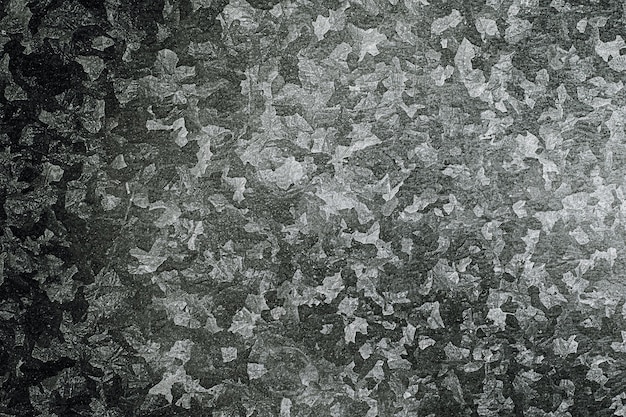The image features an abstract, hazy scene primarily in shades of black and white, with subtle hints of green that give the darker areas a greenish tint. The composition appears to resemble a lawn viewed from above, scattered with what look like numerous white bags, possibly resembling strewn garbage or fallen leaves, lending it an old and faded appearance. The overall texture is flat, with the abstract patterns evoking a sense of leaf-like forms layered over one another. The image is approximately four inches wide by two inches tall, and devoid of any text or clear elements, yet the scattered pattern of colors creates a distinct, mesmerizing effect that captures and holds the viewer's attention. This intriguing mix of textures and shades contributes to its ambiguous, timeless quality, making it reminiscent of both a weathered photograph and a faded painting.